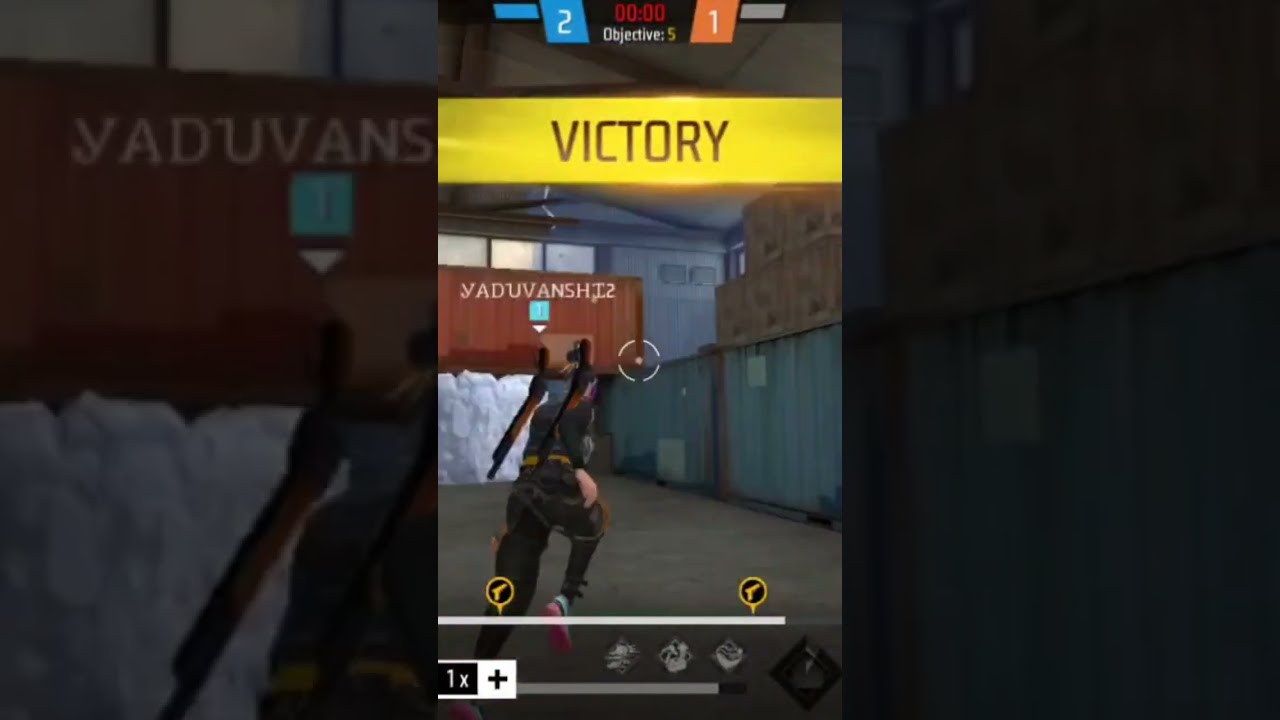The image is a detailed screenshot from a video game, likely taken from a mobile device. The central focus is a female character dressed in black pants, a black long-sleeved shirt, and vibrant hot pink shoes. She is running on what appears to be an asphalt surface in a warehouse-like environment, equipped with two shotguns strapped to her back. The scene is set amidst large shipping containers in various colors: blue on the right and reddish-orange on the left.

At the top of the screen, a prominent golden-yellow banner with black text reads "Victory," indicating a win in the game. Additional UI elements are noticeable: the score showing the blue team with two points and the orange team with one, indicating the match is over. The crosshair is centered on the screen, implying the player's aiming focus. The bottom section displays the life bar, health indicators, and other relevant game icons. The image is rich in colors, including black, white, pink, yellow, gray, orange, red, and blue, contributing to the vibrant, immersive gaming experience. The overall zoomed-in perspective emphasizes the intense and detailed nature of the game.